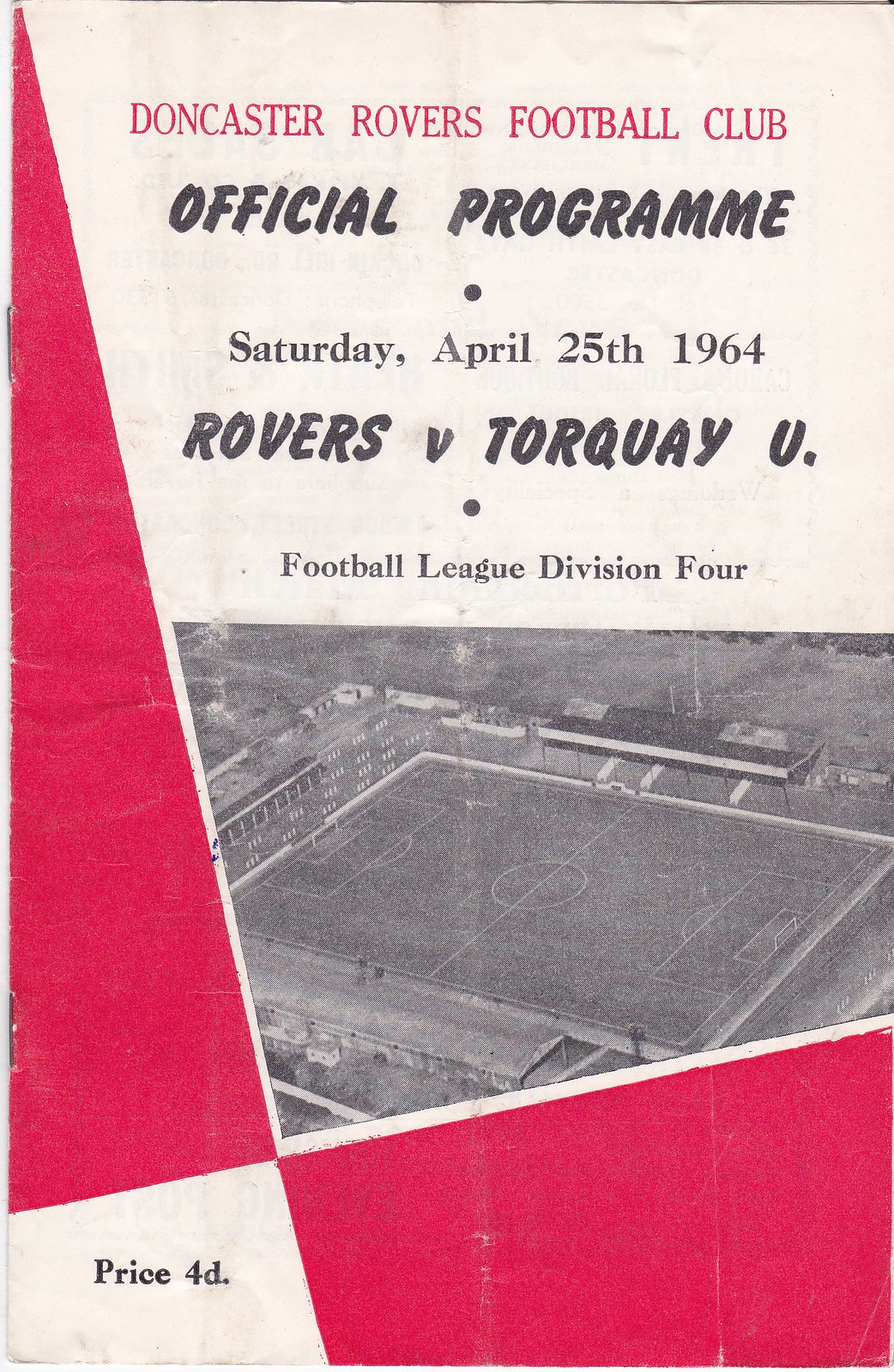The cover of this old-time British football program for the Doncaster Rovers Football Club, dated Saturday, April 25, 1964, prominently features red text at the top stating the club's name. Below this, in black text, it reads "Official Program" followed by a black dot. The matchup is specified as "Rovers vs. Torquay U" with another black dot beneath it, and the league is noted as "Football League Division IV." At the very bottom left, it mentions the "Price 4D." The cover has a striking geometric design with a red triangle along the diagonal left side and another red shape along the bottom right, intersecting over a white area. The central part of the cover displays a black-and-white aerial photograph of the soccer stadium, showcasing the field positioned horizontally across the image.